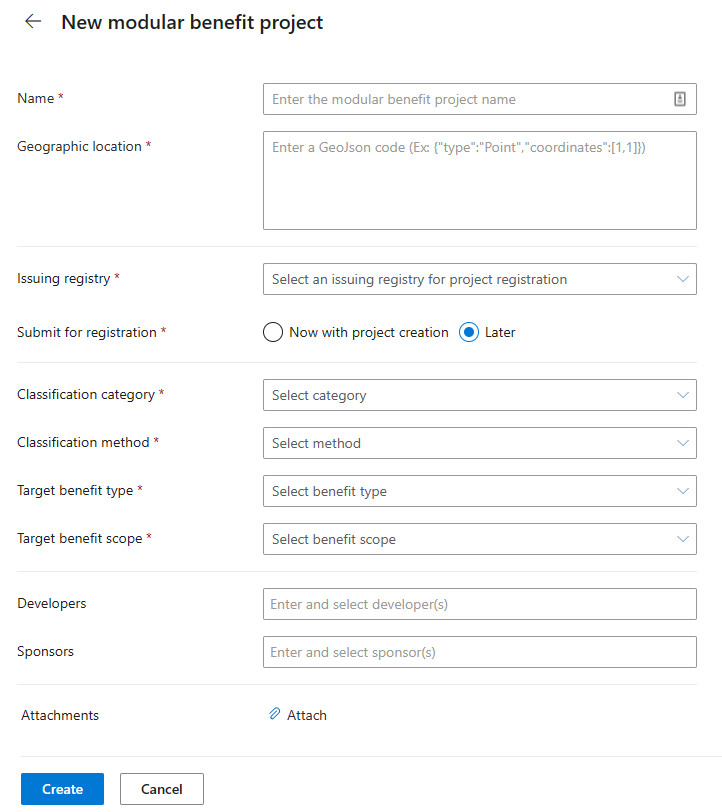The image depicts a user interface for registering a new modular benefit project. The interface is set against a clean, white background and is detailed with various fields and dropdown menus, each described below:

1. **Header Section:**
   - **Left Arrow:** Positioned at the top of the interface, likely for navigation to the previous page.
   - **Title:** "New Modular Benefit Project" prominently displayed.

2. **Name Field:**
   - **Label:** "Name" with an asterisk, indicating a required field.
   - **Input Box:** A text input area with a small square on the right-hand side.

3. **Geographic Location:**
   - **Label:** "Geographic Location" with a red asterisk, signifying it as a mandatory field.
   - **Input Box:** Another text box for entering geographic data, accompanied by an instruction to enter a GeoJSON code (example provided: `type point coordinates [1.1]`).

4. **Issuing Registry:**
   - **Label:** "Issuing Registry" with an asterisk.
   - **Dropdown Menu:** A box for selecting the issuing registry for project registration, indicated by a downward-facing arrow.

5. **Submit Button:**
   - **Button:** "Submit for Registration" in red, encased in a black circle, indicating the action to submit the project for registration.

6. **Project Creation Note:**
   - **Note:** "Now with project creation," possibly indicating a new or additional feature.

7. **Save for Later Option:**
   - **Option:** Represented by a blue checkmark, for saving the form to complete later.

8. **Classification and Category:**
   - **Labels and Dropdown Menus:**
     - "Classification Category" (with a red asterisk) and a corresponding dropdown menu.
     - "Classification Method" (with red highlights) and a dropdown menu for selecting the method.

9. **Target Benefit Details:**
   - **Labels and Dropdown Menus:**
     - "Target Benefit Type" with a select dropdown menu.
     - "Target Benefit Scope" with a select dropdown menu.

10. **Developers and Sponsors:**
    - **Labels and Input Boxes:**
      - "Developers" with fields for entering and selecting developers.
      - "Sponsors" for entering and selecting sponsors.

11. **Attachments:**
    - **Label:** "Attachments" along with a paperclip icon.
    - **Attach Button:** For uploading documents.

12. **Control Buttons:**
    - **Create Button:** A blue button labeled "Create."
    - **Cancel Button:** A white button labeled "Cancel."

This detailed caption outlines the various fields and options available for creating and registering a new modular benefit project.